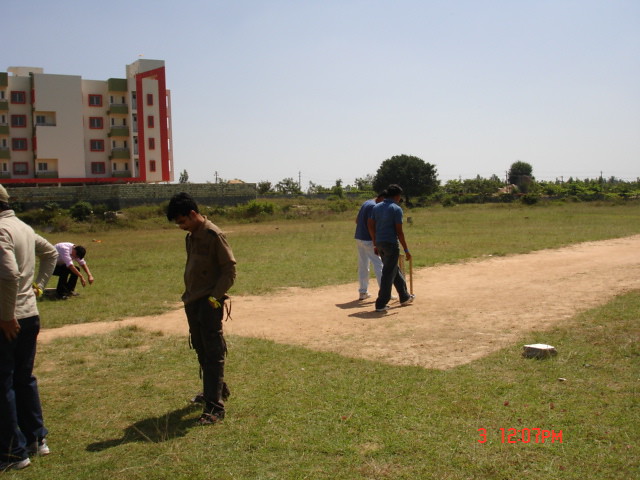In this square image, a group of individuals is scattered across a large grassy expanse mixed with dirt patches, possibly a sporting field for baseball or cricket. Dominating the scene in the upper left-hand corner is a tall condominium or hotel, roughly five stories high, made of white stone with yellow and red outlines. The top of the picture reveals a clear blue sky, while the middle section frames a couple of distant trees. Cutting across the field towards the right is a rectangular dirt path. Two men are seen walking along this path, one holding what appears to be either a cane or a bat in his right hand. On the left side of the field, another man stands with his hands in his pockets, gazing down at the grass. Further to the left, another man's body is partially visible, facing away from the camera with his face cut off, while yet another man in the far background might be either hunched over stretching or sitting on a bench. The timestamp at the bottom reads "3, 12:07 p.m." in red letters.